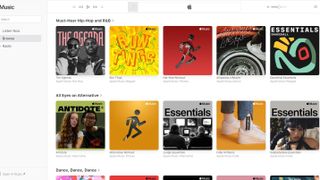This is a very blurry image of a music selection page from Apple's platform, likely the homepage. The image is so indistinct that zooming in doesn't reveal much detail beyond the recognizable Apple logo. The visible content appears to be a collection of curated playlists and essentials. Some of the highlighted sections seem to feature themes like car tire essentials and perhaps a playlist titled "Antidote." There's also a mention of a person with something in their sock, indicating another curated essential playlist. The page seems to be designed for navigation and song selection, tailored for users accessing it via an iPhone or iPod, hinting at Apple's emphasis on integrated digital music experiences over traditional mp3 players. Despite the blurriness, the image conveys the familiar look and feel of Apple's user interface, focused on providing curated music collections.